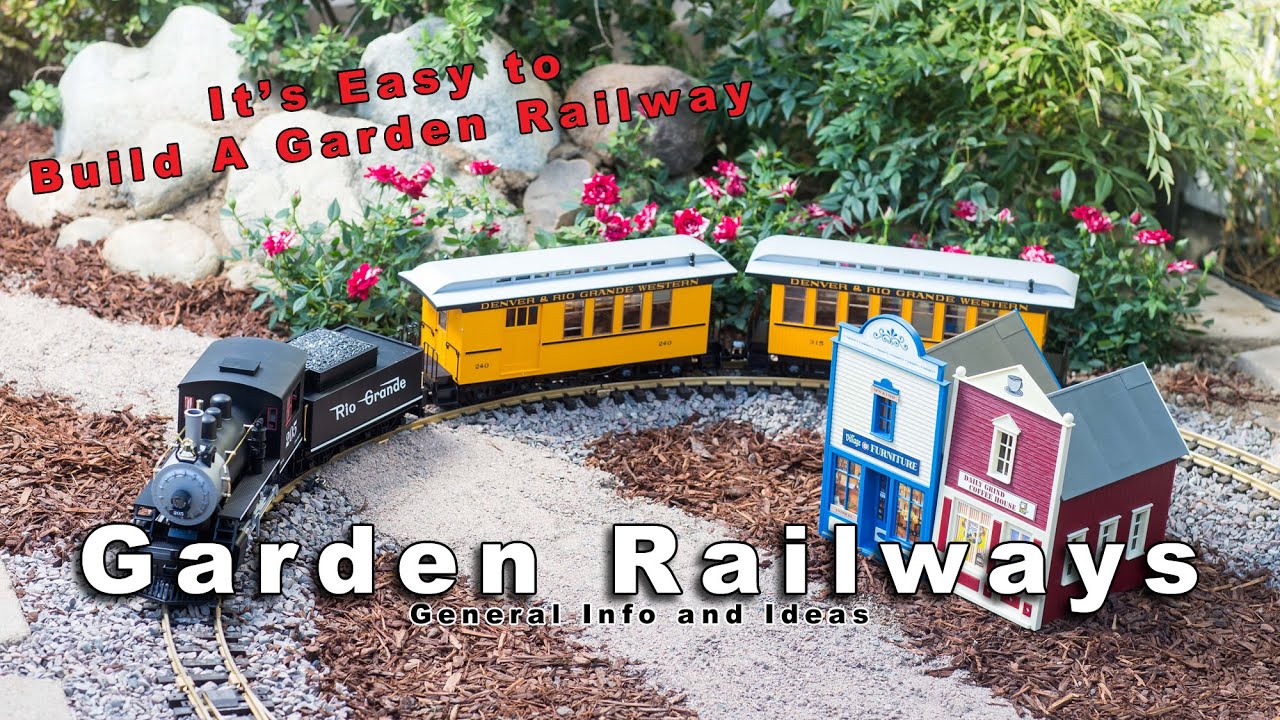The photograph showcases a vibrant garden railway scene, complete with a detailed toy train set nestled amidst a lush garden bed. At the top, bold red text declares, "It's easy to build a garden railway," while the bottom of the image provides "General info and ideas" about garden railways. 

The train itself is a charming model, with a black engine at the front labeled "Rio Grande" and two yellow cars trailing behind. The train navigates a circular track surrounded by bark, gravel, and stones, with ample room to add more cars to the back if desired. Flanking the track are two quaint buildings: a furniture shop in blue and white and a coffee shop in dark red with white accents and a pointy roof. 

In the background, larger rocks and green foliage, including some pops of pink flowers, add to the garden's appeal, creating a visually appealing and immersive miniature railway experience.